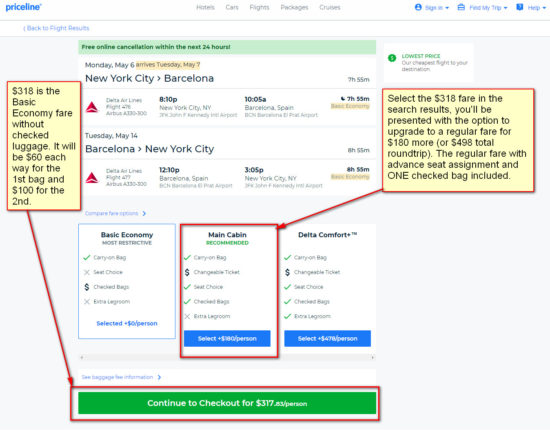**Detailed Caption:**

This image is a cropped and edited screenshot of the flight booking page on Priceline.com. The top left corner of the web page features the Priceline logo in blue font. At the top center, a navigation bar displays options for "Hotels," "Cars," "Flights," "Packages," and "Cruises" in grey font. On the top right, there are blue icons and words for "Sign In," "Find My Trip," and "Help."

The main body of the webpage is grey. On the top left, the text "Back to Flight Results" is displayed alongside a left-pointing arrow. Below this, a large white box is positioned at the center of the page. A green banner at the top of this box reads "Free Online Cancellation within the next 24 hours." Beneath this banner, there are flight details displayed. The upper left section of the details area shows the day and date, as well as the departure and arrival airports.

On the left side of the screenshot, there is an edited red box with an arrow pointing downward, connecting the box to a green bar at the bottom that says "Continue Checkout." This bar includes details about the flight's price.

At the bottom portion of the web page, three boxes labeled "Basic Economy," "Main Cabin," and "Delta Comfort" are shown. The "Main Cabin" option is selected, highlighted by a red box edited around it, and there is an arrow pointing from the right side box to the "Main Cabin" box. The red box includes further instructions that say, "Select the $3.18 fare in the search results," along with more specific guidance.